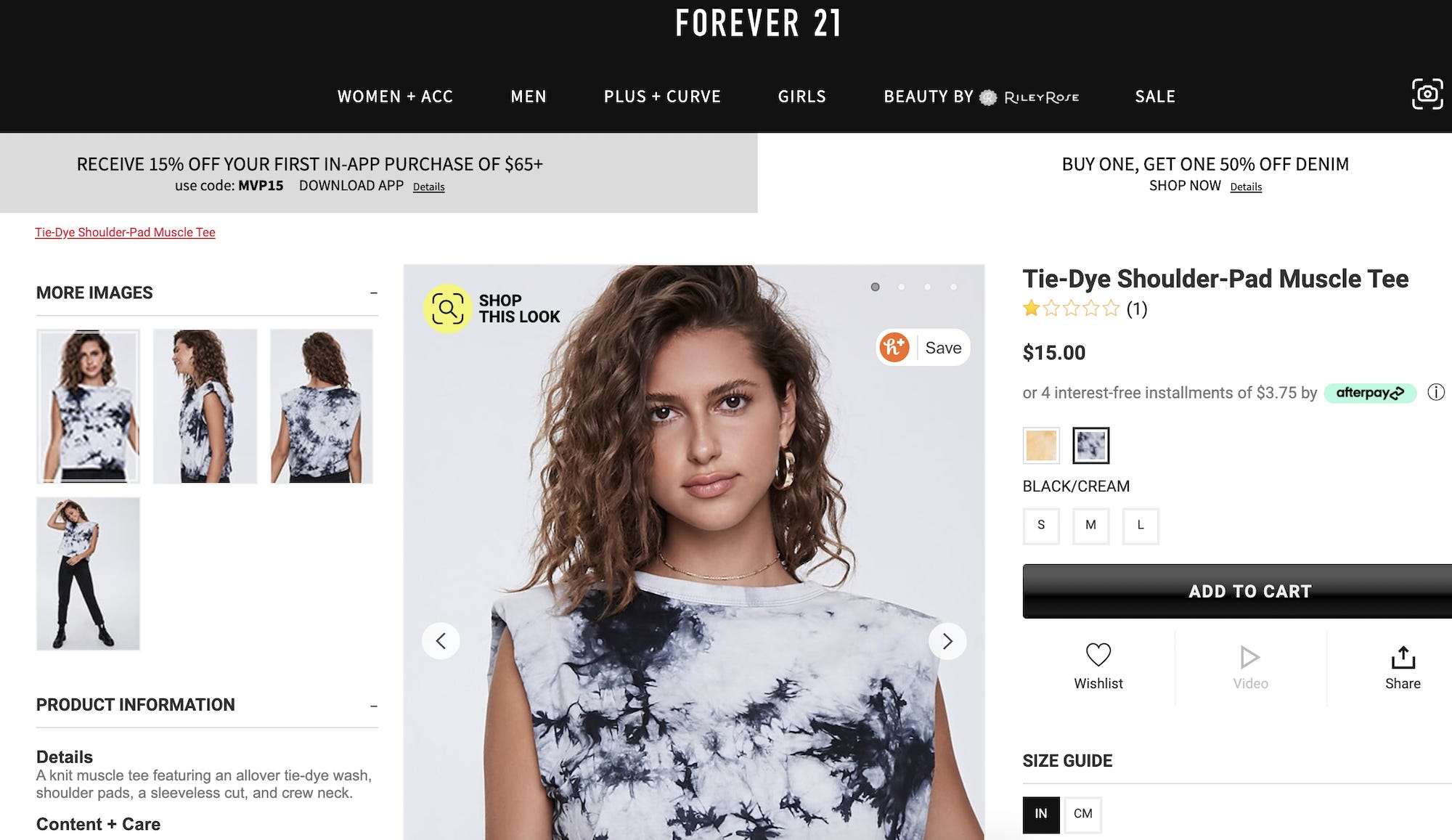The image showcases the Forever 21 website interface. Dominating the top section is a prominent black header box with "Forever 21" emblazoned in white text. The navigation menu underneath is clearly laid out with categories: Women, Accessories, Men, Plus and Curve, Girls, Beauty by Riley Rose, and Sale. 

Beneath this, a smaller gray notification box announces a limited-time offer: "Receive 15% off your first in-app purchase of $65 or more. Use code MBP15. Download the app for details." Adjacent to this, another promotion advertises a "Buy One, Get One 50% off denim" deal.

The main content of the image focuses on a product listing for a tie-dye shoulder pad muscle tee. The product is modeled to display multiple angles, including the front, back, and side views. The description notes that the tee is a knit fabric with an all-over tie-dye wash, featuring shoulder pads, a sleeveless cut, and a crew neckline. The specific color variations available are black and cream tie-dye, and oatmeal.

Notably, the product has received a one-star rating and is priced at $15. The interface includes options to add the item to the cart or wish list, watch a product video, share the product, and consult a size guide, which provides measurements in both inches and centimeters.